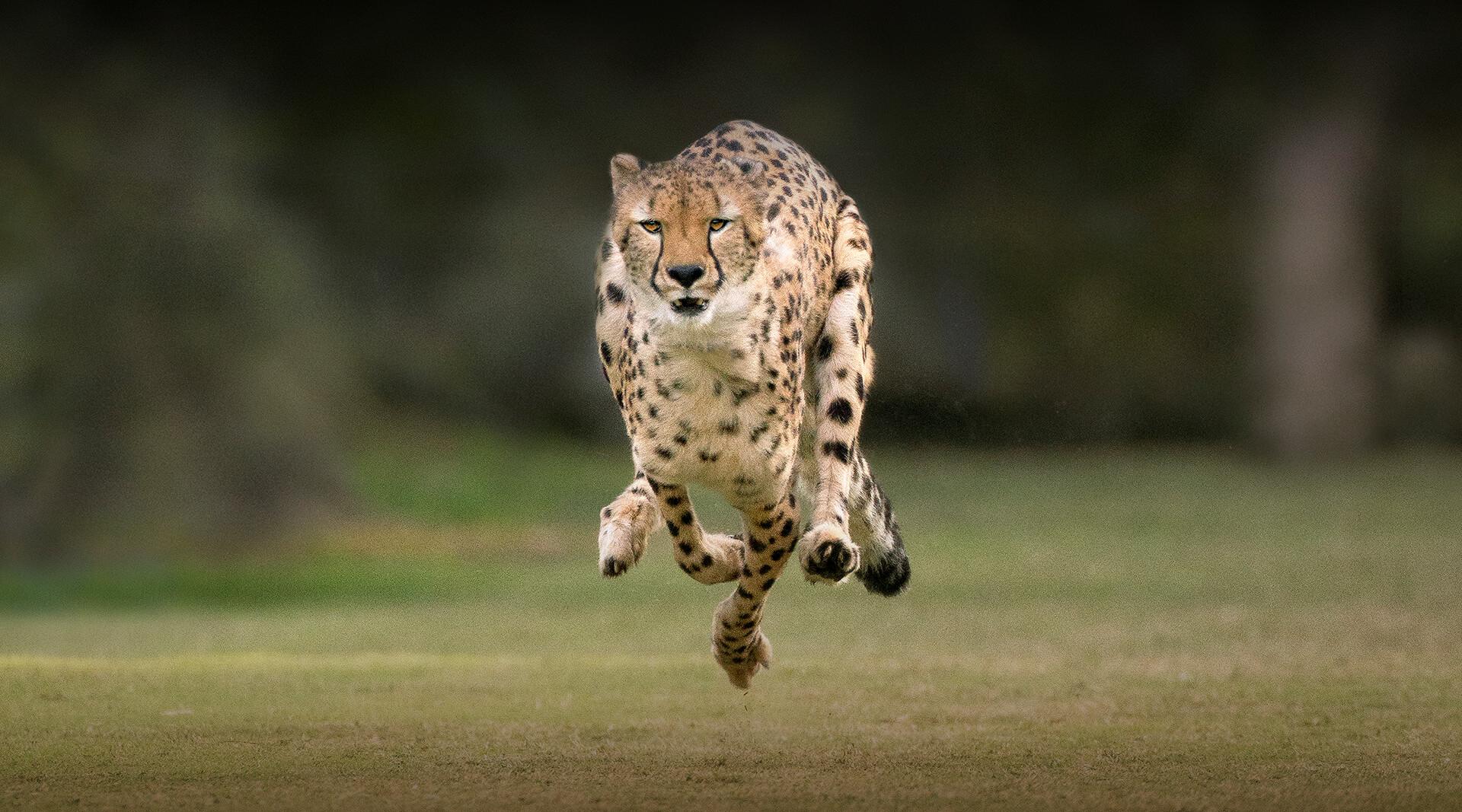In this dynamic action shot, a cheetah is captured mid-run, seemingly leaping through the air with all four legs off the ground. The front left leg trails slightly behind, while the front right leg is closer to the ground, suggesting it has just pushed off from these legs. The back legs are tucked forward, enhancing the sense of motion towards the viewer. The cheetah's alert eyes, a pale yellowish tan framed by black markings, stare directly at the camera, its mouth closed in focus. The animal's characteristic golden-brown fur adorned with black spots is vividly detailed, transitioning to a lighter white underbelly that widens slightly before darkening towards the spine. Its tail extends straight back, balancing its motion. The cheetah's tan face, small black-tipped nose, and dark black paw pads add to the visual richness of the image. The background is a blur of green grass and indistinct trees, emphasizing the speed at which the cheetah races across the smooth terrain. This perfectly timed photograph showcases the grace, power, and beauty of the cheetah in its natural habitat.